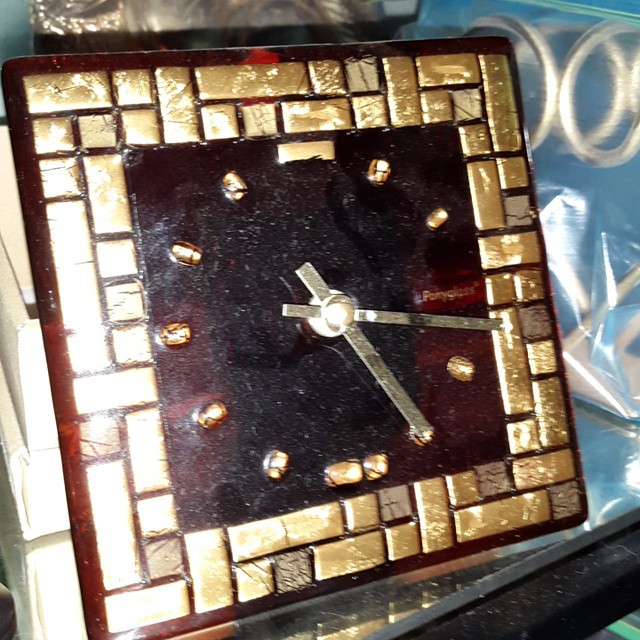The image depicts a highly decorative, square-shaped analog clock prominently displayed indoors. The clock features a striking border composed of two layers of variously-sized gold blocks, interspersed with golden squares and rectangles. Each block is set against a black backdrop, contrasting sharply with the intricate gold pattern. The clock face itself is black, framed by smaller gold dots that represent the hour markers, from 1 through 11, with rectangles specifically denoting the 12 and a split rectangle for the 6. The clock hands are thick, rectangular pieces of silver metal. Notably, there is a gold block at the top with text, while on the right side, 'party glass' is visible in gold text. Surrounding the clock are several silver circular objects encased in a clear plastic bag, all situated on a flat, see-through glass shelf. The surroundings hint at an artisanal or antiquarian setting, enhancing the clock’s unique and handcrafted appearance.